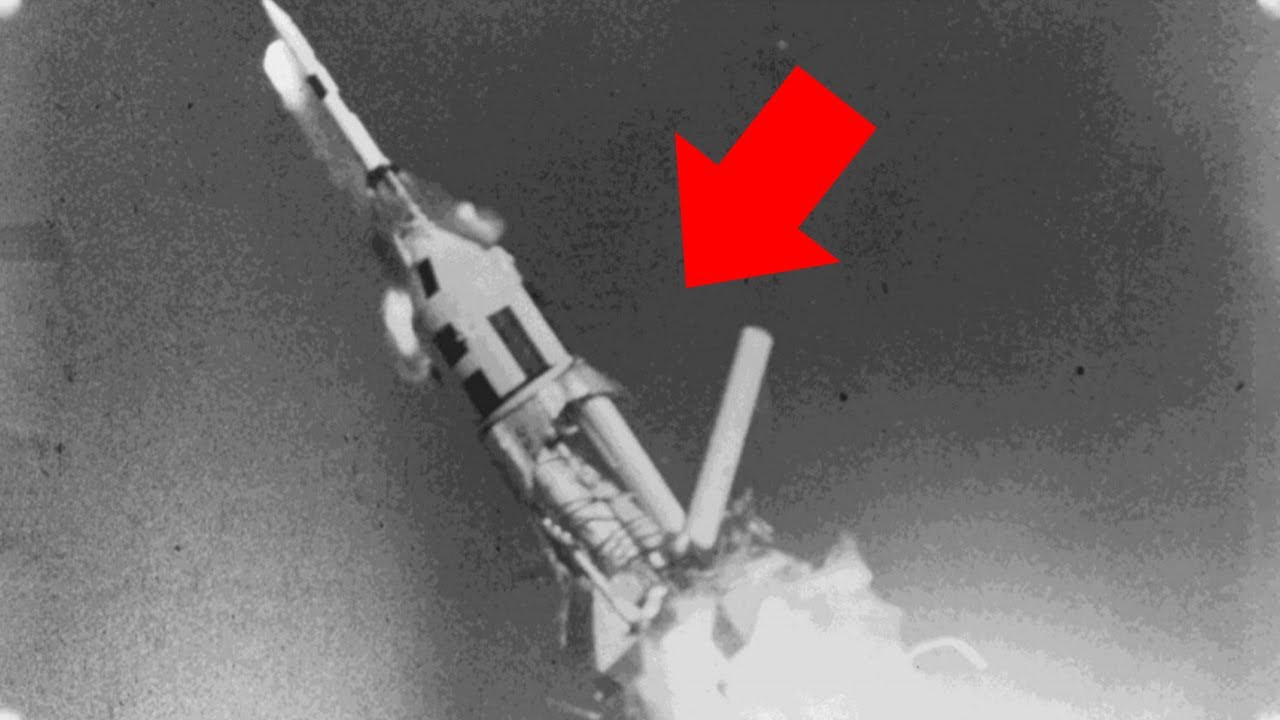The black-and-white image, likely from the 1950s or 1960s, depicts a dramatic rocket launch, captured from a distance using a telescopic lens. The rocket, predominantly white with some black features and doors, is seen blasting off at an angle towards the left against a grayscale background. A large red arrow points to a specific area on the body of the rocket, drawing attention to the scene. At the base of the rocket, flames and an explosion are visible, with tubes visibly bursting, suggesting a critical malfunction. Despite the explosion, the upper part of the launch vessel, including the pod and capsule, appears to be ejecting safely and exiting the danger zone, indicating the possible activation of a safety device. The photograph shows a cylindrical body that widens as it nears the jet engines, which are engulfed in fire, propelling the rocket skyward. The image is distressed and pixelated, adding to its vintage and somewhat ambiguous nature.